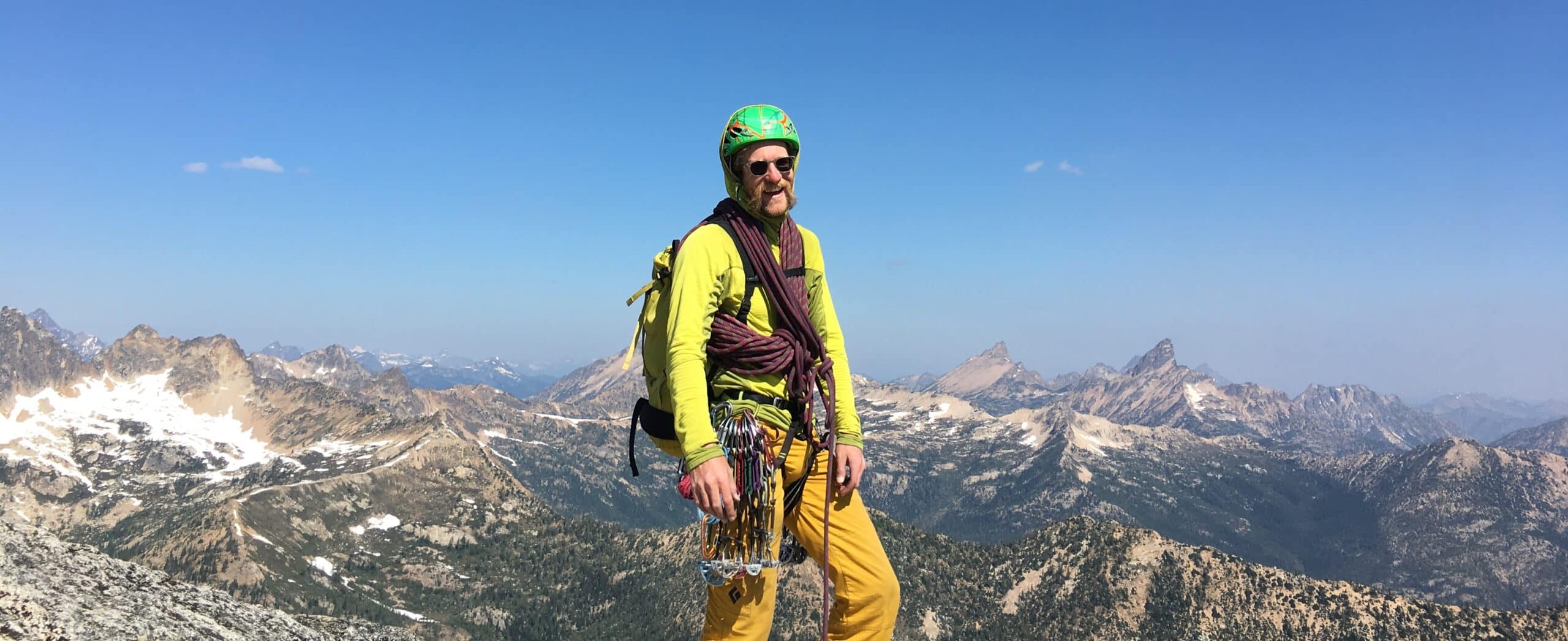The image is a horizontal photograph featuring a mountain climber standing prominently in the center. The climber is facing forward with a slight turn to the right, wearing a green helmet, sunglasses, and sporting a mustache. He is dressed in a yellow climbing suit comprising a shirt and orange-yellow pants, with a purple scarf around his neck. He has a belt equipped with climbing tools, including various hooks, hanging down over his right thigh and ropes draped around his body. A large yellow backpack is strapped on his back. The background reveals a panoramic view of mountainous terrain; the closer hills to the bottom right are covered with thick trees, while the more distant peaks feature a mix of snow patches and bare rock, stretching up to meet a clear blue sky dotted with a few small white clouds.